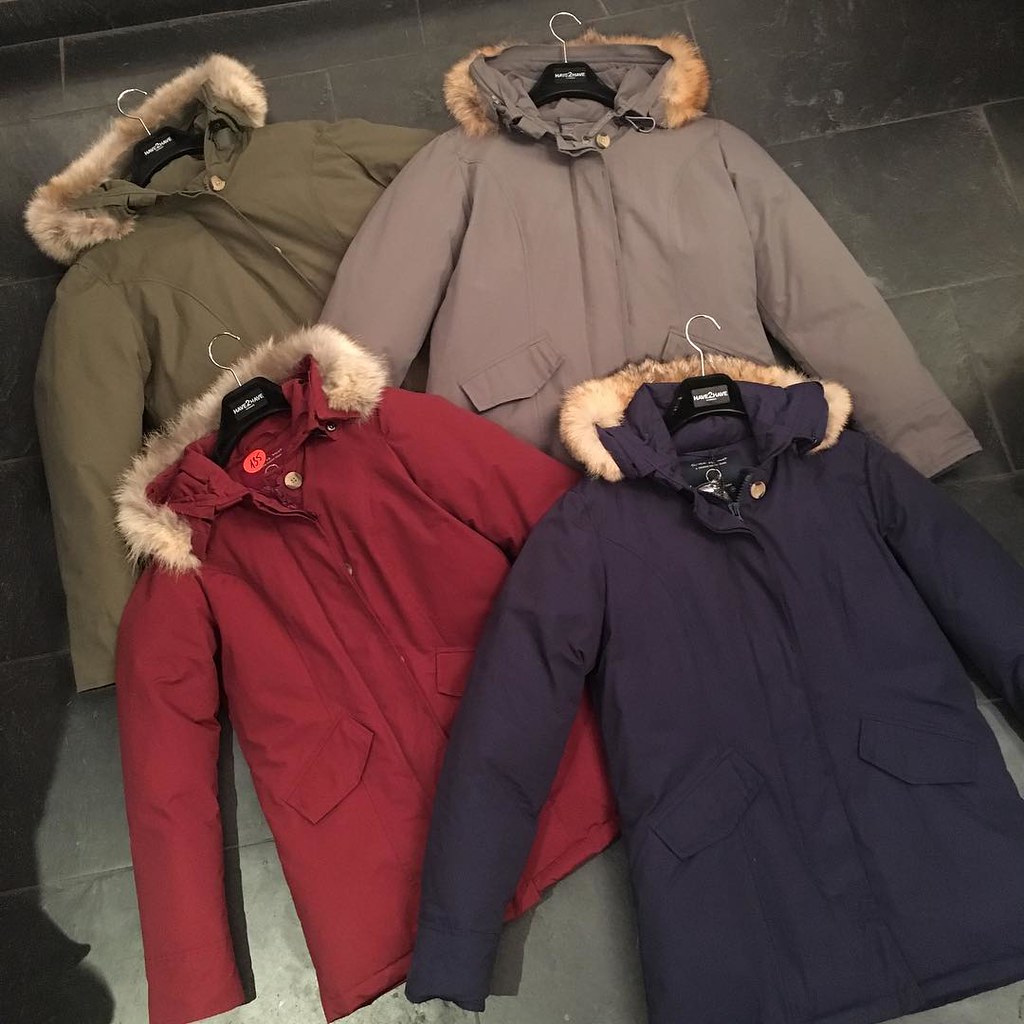This overhead photograph captures four winter jackets laid flat on a large, black slate-tiled floor with rectangular patterns, which appear to continue slightly up the wall in the top left corner. Each jacket is a similar style featuring two front pockets, zippers, front buttons, and hoods lined with faux fur. All four jackets are on black hangers. Starting from the top left, the jackets are olive green, light gray, dark red (featuring a tag that reads number 35), and navy blue. The lighting overhead creates a shadow you can glimpse on the left-hand side, possibly cast by the photographer. The jackets vary slightly in size, with the top ones appearing marginally larger.